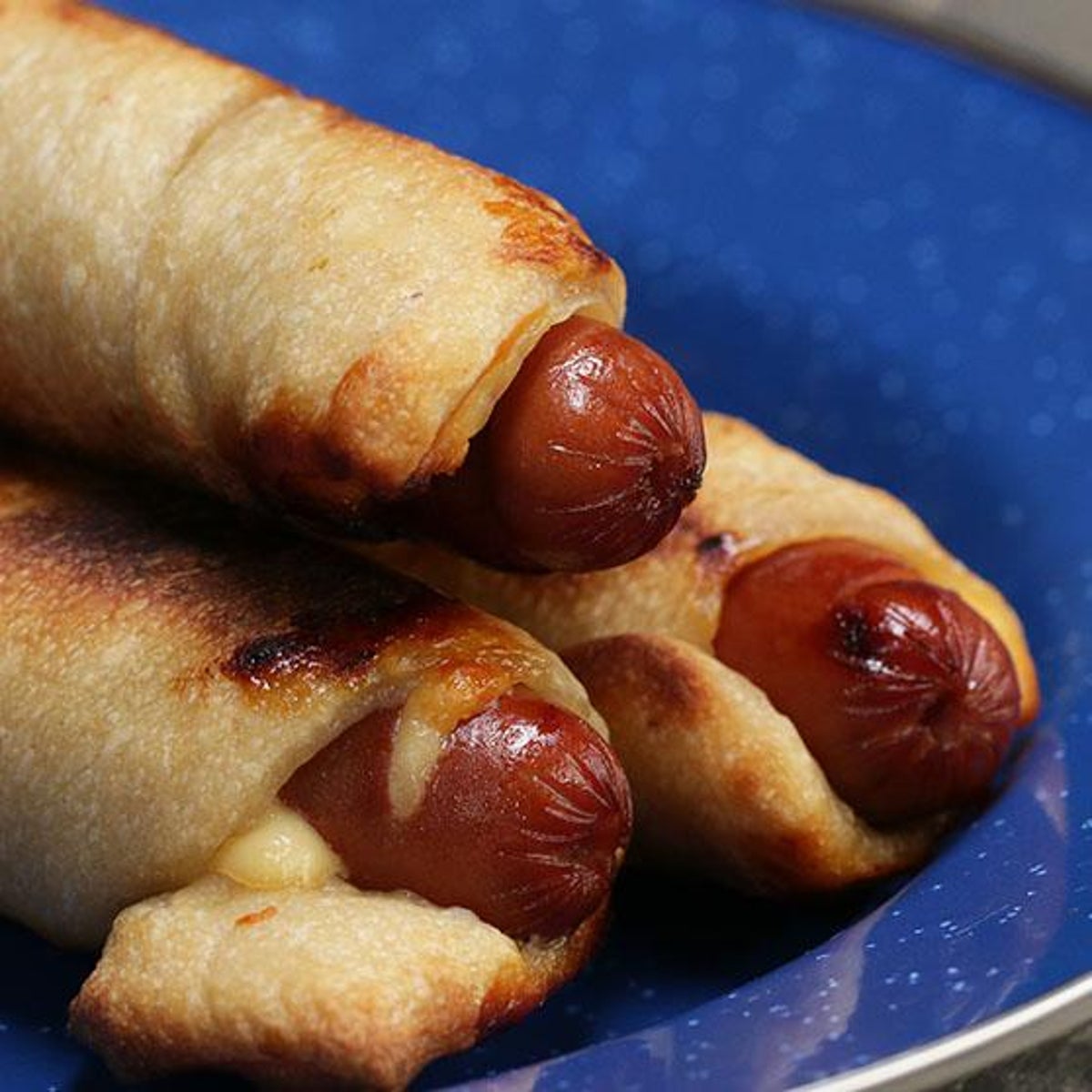The photograph showcases a close-up, professionally-shot image of three hot dogs wrapped in crescent roll pastry, often called pigs in a blanket. The hot dogs are nestled with just their ends emerging from the golden-brown, slightly crispy pastry, some areas of which are darker due to light charring. This trio of hot dogs is stacked in a pyramid formation—two at the bottom supporting one on top—on a blue metal plate with subtle white specks, resembling a pattern of baby blue dots. The plate, which has the appearance of a shallow bowl, is partially out of focus, especially beyond the immediate area of the stacked hot dogs, drawing attention directly to the detailed texture and color of the crescent rolls and hot dogs. The hot dogs exhibit an appealing reddish-brown hue, indicating they are thoroughly cooked. The entire setup hints that the image could be intended for a cookbook or a food magazine.